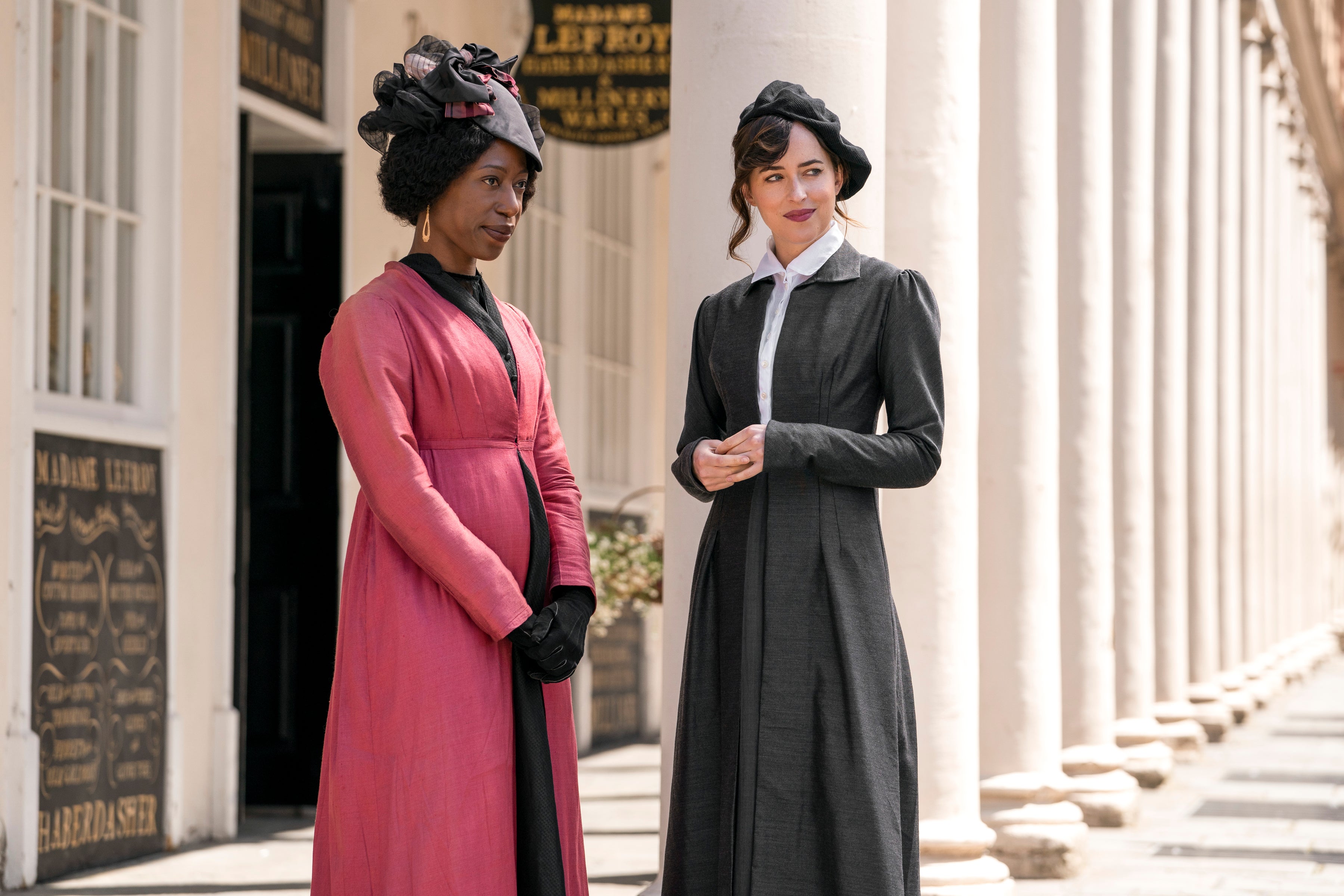The image depicts two women standing side by side in front of a grand white cement building with large, square-topped columns receding into the background. Both women are elegantly dressed in long coats and hats. The woman on the left, who has dark skin, is wearing a red dress under a pink overcoat and has black gloves on. Her black hat is adorned with white and reddish flowers. The woman on the right, with lighter skin, is dressed in a white collared shirt with a thin long coat and a small black cap. They are both looking towards the right. Nearby, a sign with pictures, possibly of flowers, hangs to the left above an entranceway that has a black section above it. There are also some subtle green leaves from a flower pot visible between them. The photo appears to be taken outdoors during daytime.